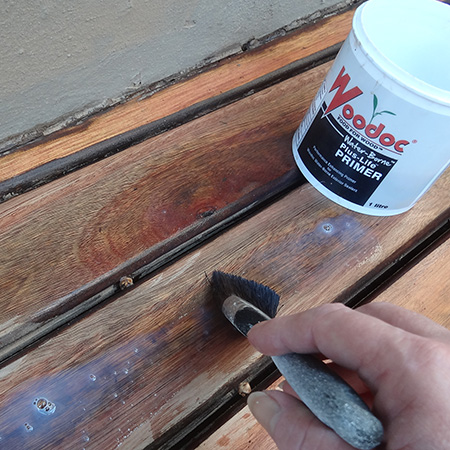In this detailed close-up image, the main subject is a hand using a wooden paintbrush to stain a surface that resembles a wooden table, floor, or deck. The wood has a dark, cherry-like finish, and the brush is applying a milky liquid, which is likely a stain or paint. To the right of the hand, there is a white container, which could be made of plastic or metal. The container has red text on it that reads "WOODOC." Between the "O" and the "D," a small green sprout is subtly illustrated. Below this text, there is a black box with white capital letters that seems to say "PLASTER PLUS-LIGHT PRIMER," though the exact wording is somewhat unclear. The scene captures the meticulous process of wood staining, highlighting the precision and care involved.